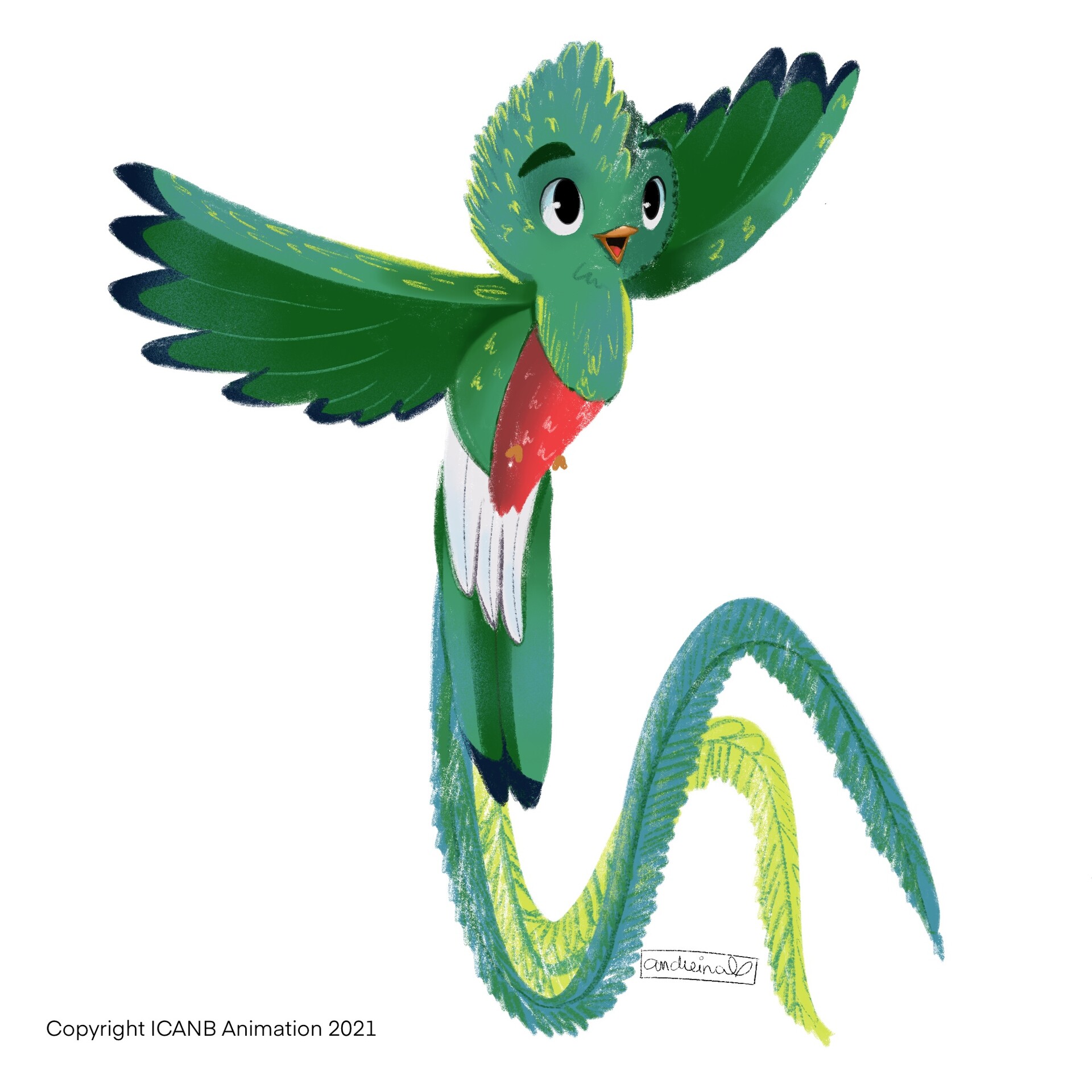The image showcases a vibrant, painted or drawn bird that appears to be a fantastical blend of dragon and bird elements. The bird stands facing the viewer with its wings spread wide, gazing upwards towards the sky. Its primary color is green, with striking blue tips on its wings and additional white accents. Wrapped around its neck is a red handkerchief, decorated with a subtle floral pattern, which covers the bird’s stomach.

The bird's tail is elaborate, beginning with short white feathers, transitioning into green swirls, and extending into two prominent, elongated feathers—one yellow and one matching the bird’s green. At the bottom left corner of the image, a copyright notice reads "ICANB Animation 2021." Additionally, a rectangular tag bears the name of the artist, "ANDIE INALL." This artwork is a detailed and imaginative illustration, ideal for those who appreciate intricate and whimsical designs.